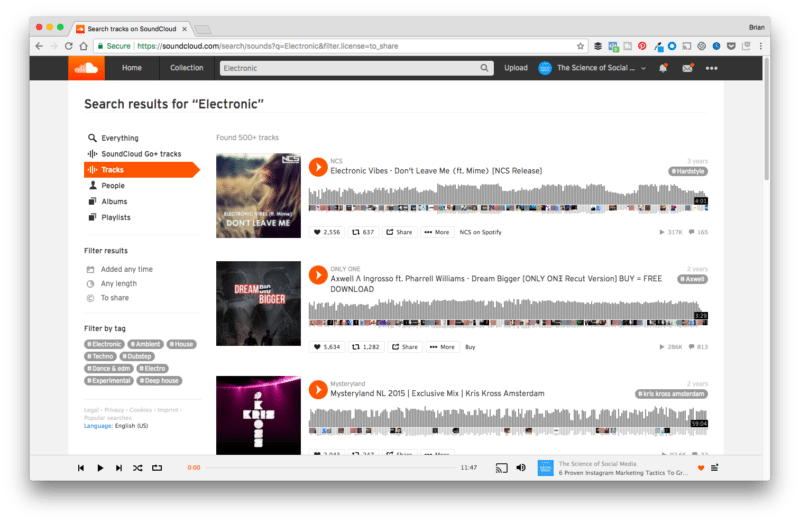This screenshot from a Mac displays the SoundCloud website. In the top-left corner of the browser window, the familiar red, yellow, and green buttons for closing, minimizing, and maximizing are visible. To the right of these buttons is the browser tab for the current site.

Below the browser's toolbar, there is a navigation bar featuring a left arrow for going back, a right arrow for going forward, an undo icon, a refresh icon, and a home icon. The address field is positioned centrally in this toolbar, flanked by several function icons on its right side.

The main webpage shown in the screenshot is SoundCloud. In the upper left corner of the SoundCloud interface, there is an orange square with the white SoundCloud logo. Directly to the right, there is a black border containing the options "Home" and "Collection," followed by a search field. Further right, there are options to upload content, view the user account, check notifications, and access additional options through a button featuring three dots.

The main content area of the webpage has a white background. In the upper part of this area, "Search results for electronic" is written in black font. A side pane on the left displays several options: "Everything," "Tracks," "People," "Albums," and "Playlists." The "Tracks" option is currently highlighted in orange, indicating the selected category. Below this, there are options for filtering results, including "Filter by Tag." To the right, within the main display area, three SoundCloud audio options are available for playback.

Overall, this screenshot provides a detailed look at the SoundCloud search results interface with a focus on electronic music tracks.